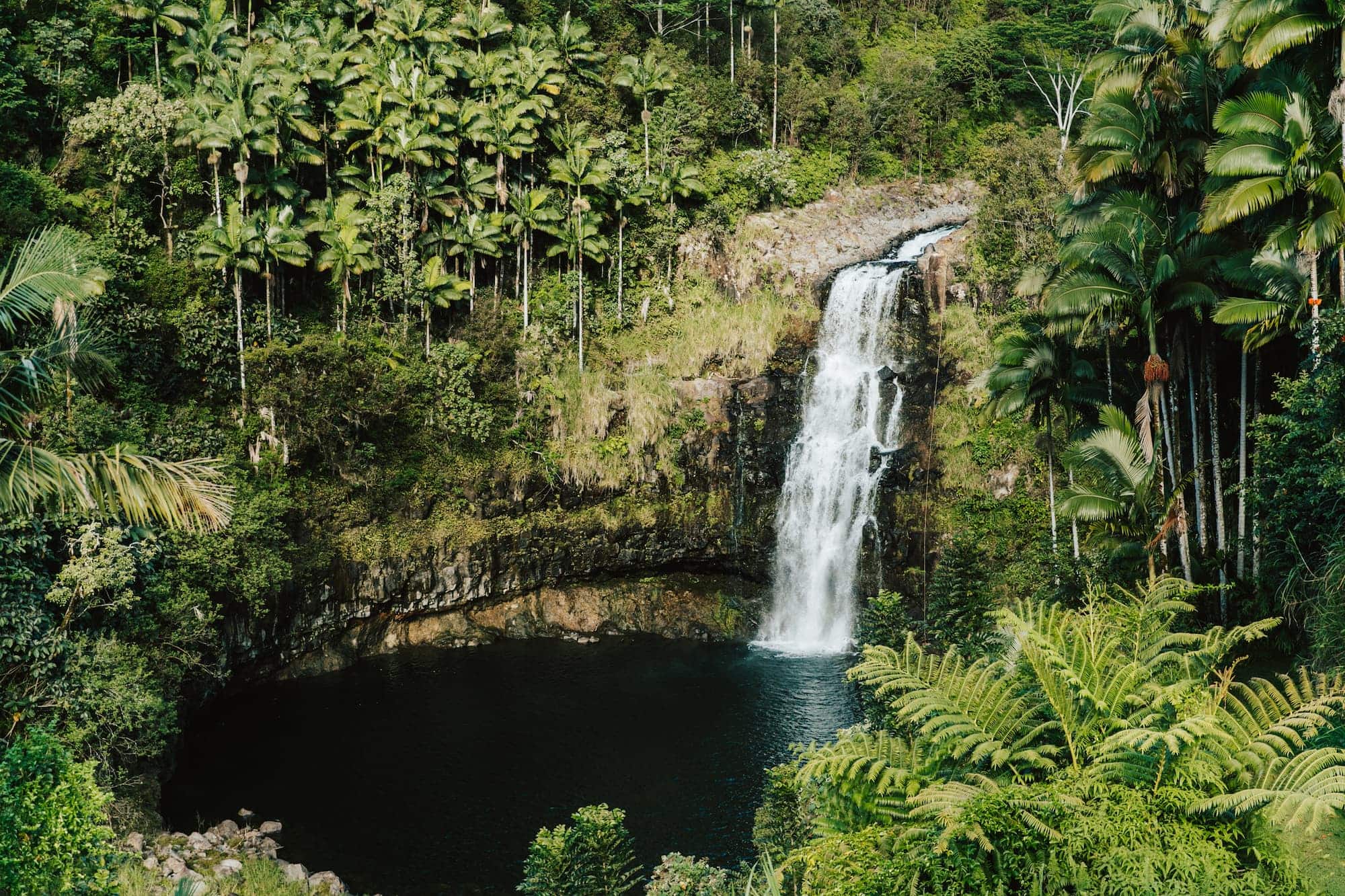A vivid outdoor photograph captures a pristine jungle scene with an impressive waterfall slightly to the right of center. The waterfall cascades down a steep, cliff-like hillside, creating a striking white streak against the lush, green backdrop. The waterfall empties into a tranquil, dark blue lagoon located in the lower part of the image. The stillness of the water allows for a clear reflection of the rocks above, with subtle ripples adding texture to the serene surface. Surrounding the lagoon is dense tropical foliage, including various types of trees, palm fronds, and fern bushes. Tall palm trees can be seen both beside and above the waterfall, contributing to the dense, layered greenery that stretches across the entire background. The cliffy hillside on the upper left is also covered with more tall palm trees and a rich assortment of tropical plants, creating an immersive canopy of vegetation that obscures any view of the sky. The scene exudes a sense of untouched natural beauty, with no visible animals or humans present.